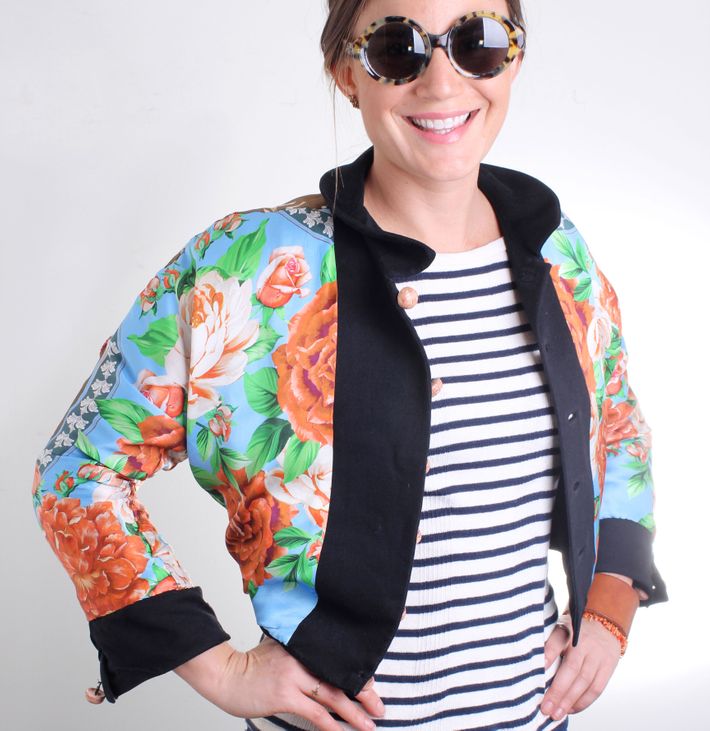In this vibrant image, a smiling Caucasian woman of European descent is captured in a close-up shot against a white background. She has fair skin and white teeth, accentuated by her pink lipstick. Adorning her face are sunglasses with a distinct cheetah-like yellow and black pattern, which also reflect the bright screen she appears to be looking at.

Her dark brown hair is neatly tied up, giving a clear view of her attire. She dons a striking, brightly colored floral jacket with a blue background, adorned with various shades of pink flowers and vivid green leaves. The jacket has navy blue sleeves, complemented by a pattern of green and white flowers near the cuffs. The coral pink buttons on the jacket stand out prominently. Beneath this, she wears a white shirt with horizontal black stripes.

Accessorizing her outfit, the woman sports an orangish bracelet along with an orange-brown leather wristband on her right hand. Additionally, she has a ring on her right ring finger and is wearing earrings, likely on both ears. Overall, her confident posture, bright smile, and colorful ensemble create a cheerful and engaging portrait.